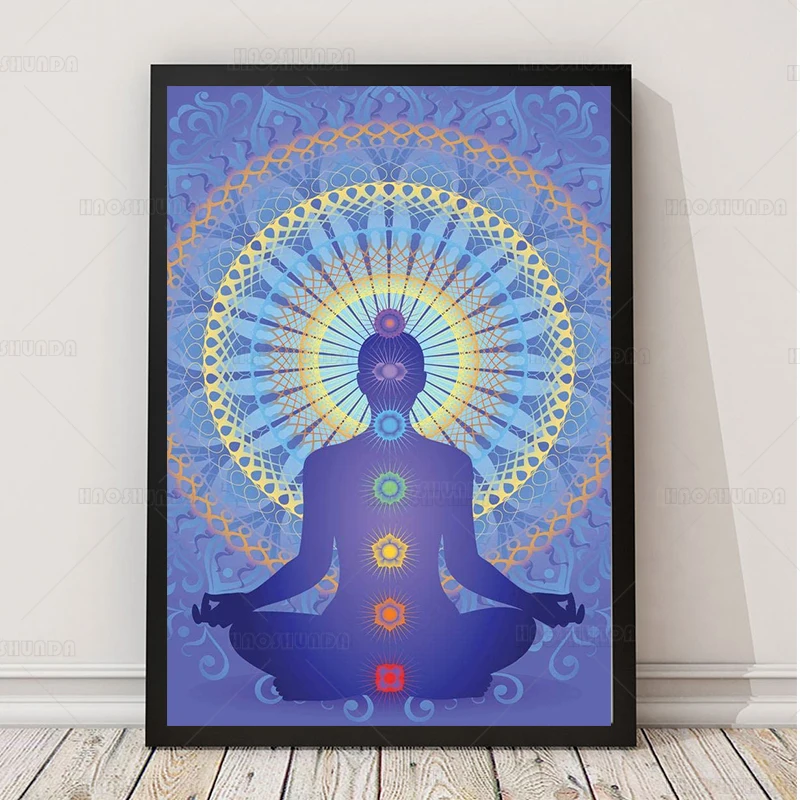A large, framed poster depicted in a black frame leans against a white or off-white wall in a living room. The floor beneath it is a distinctive white wood with subtle streaks of orange and brown. The mystical poster visually represents a person in a meditative pose, legs folded beneath them, arms outstretched with hands resting on their knees, and fingers and thumbs forming a mudra. The figure is rendered as a blue silhouette against a vibrant blue background filled with lightbulb-shaped motifs encircling the center. Surrounding the meditative figure are concentric circular weaves of orange, yellow, blue, and red. From the top of the figure's head down to the base, various chakra symbols are illustrated as round, textured orbs with radiating thorns. Notably, the head has distinct eye symbols featuring a central circle flanked by half-arrow shapes. Further down, the chakras continue with color-coded representations: a blue orb, a green one, and a triangle-shaped symbol at the abdomen resembling a house with a central yellow circle. Additionally, a star shape adorned with orange and a blue ring, followed by a red square bordered by a blue ring, mark the lower chakras. The vibrant palette includes shades of purple, blue, red, orange, yellow, green, light blue, and a hint of light purple, capturing the essence of the chakras. This framed artwork, positioned directly in the center of the room against the wall, offers a focal point that blends spirituality with colorful artistry.